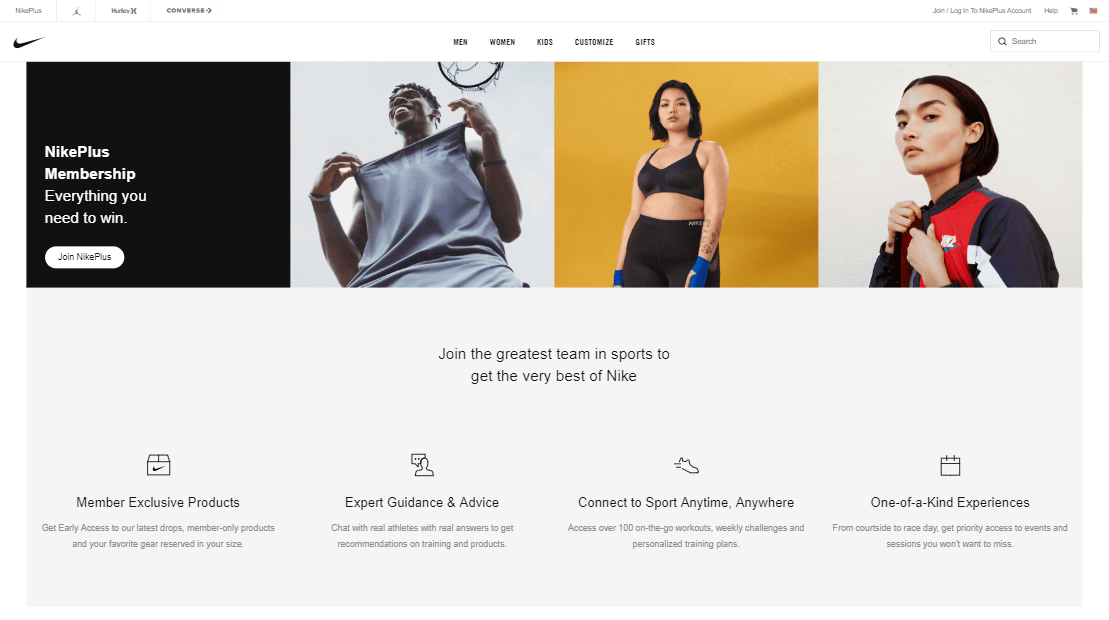This is a detailed screenshot of the Nike Plus website. In the upper left-hand corner, "Nike Plus" is prominently displayed, with a small icon of the Jordan brand next to it. Additionally, there are two more tabs; although the third one is indistinguishable, the last tab is identifiable as Converse. The main page showcases five categories: Men, Women, Kids, Customized, and Gifts. To the right of these categories is a search bar.

The content of the page itself is segmented into four distinct boxes. The first box is nearly perfectly square, black in color with white text that reads, "Nike Plus membership: everything you need to win." Below the text is a white button with black text that says, "Join Nike Plus."

To the right of this box is an image of a smiling black gentleman wearing a gray Nike shirt. The photo, taken from a lower vantage point, looks up towards him, suggesting he may be tall. He is smiling happily while pulling on his shirt to display the Nike logo. He is clean-shaven, sporting a bracelet on his left arm and possibly a watch on his right.

Next to this image is an Asian woman with her hands wrapped in blue wraps. She is dressed in a sports bra and black tights, ready for physical activity.

The final section features a woman in a red jacket with navy sleeves. She has a serious, scowling expression and her face is slightly turned to the left, showcasing the left side of her face more prominently.